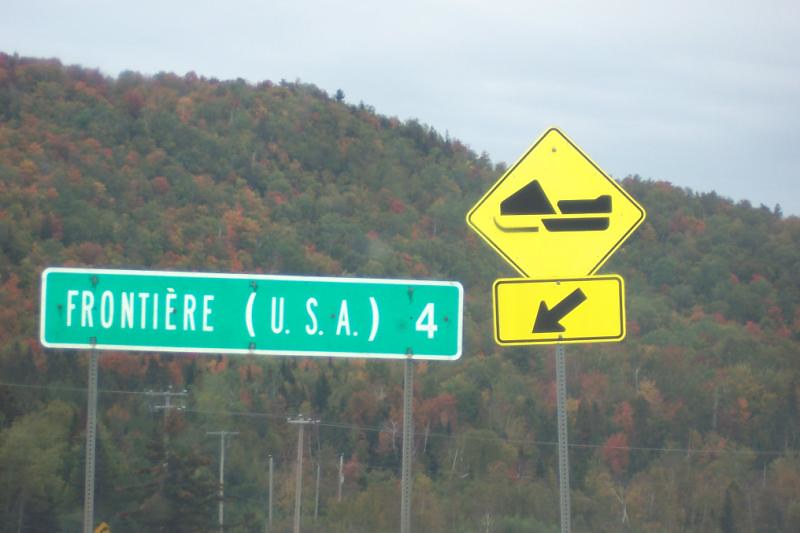This photograph captures a section of the highway featuring multiple signs and a picturesque natural backdrop. Centered prominently is a large, green highway sign with white trim. The sign reads "Frontière" (French for "Frontier"), with the accented "é" clearly visible, followed by "(U.S.A)" and "4." This indicates that the U.S. border is 4 miles away. 

To the right of this main sign, a yellow diamond-shaped sign is present, featuring an image resembling a snowmobile, likely indicating a snowmobile crossing area. Directly below, a smaller rectangular yellow sign with a black arrow points downward and to the left, providing additional directional guidance.

Behind these signs, the scenery is dominated by a majestic mountain range and a mix of green, red, and orange trees, suggesting the vibrant colors of fall foliage. Overhead, power lines are faintly visible against the natural background, adding an industrial element to the otherwise serene landscape.